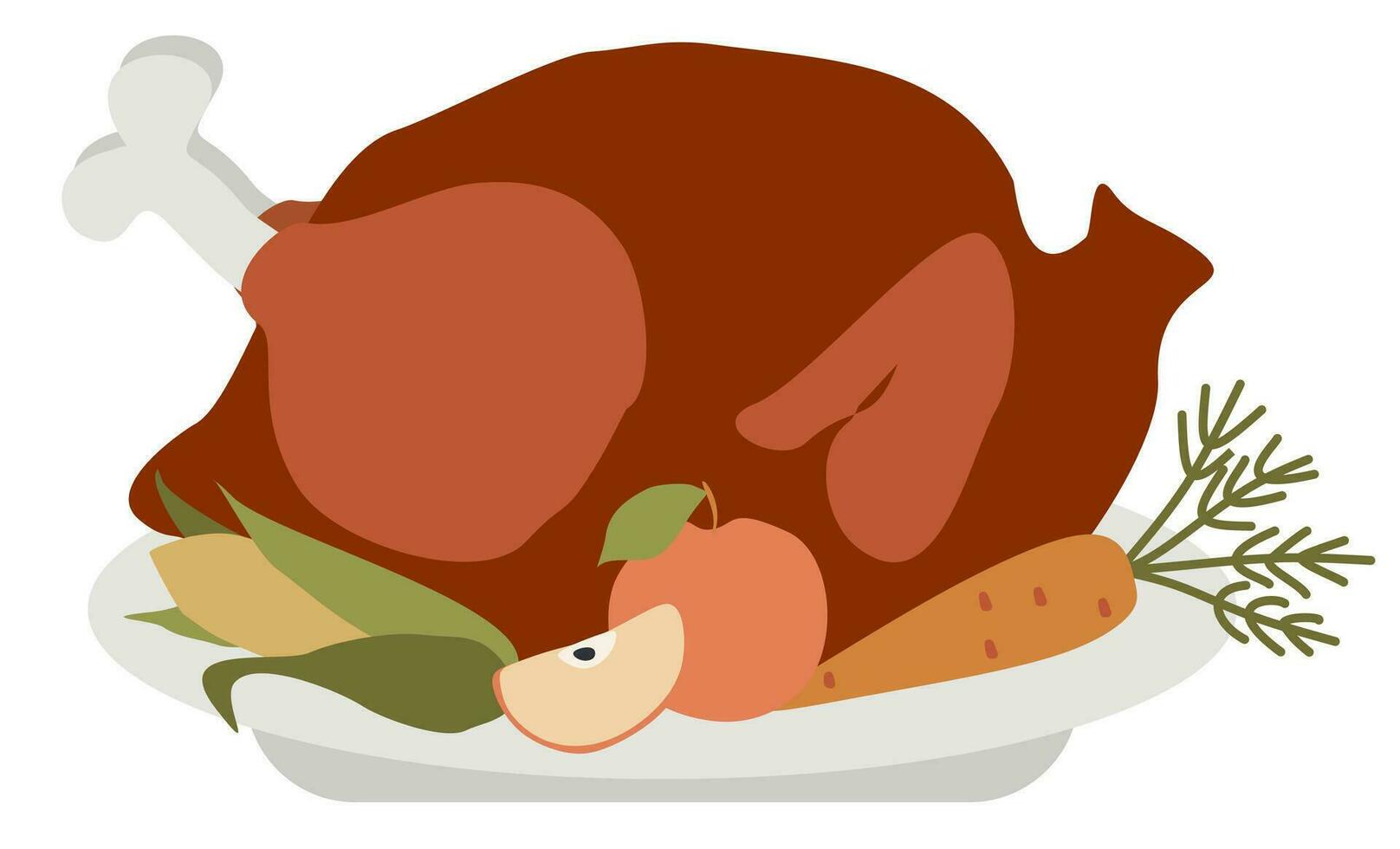This image is a computer-generated, cartoonish 2D illustration of a cooked, roasted turkey displayed on a white plate against a white background. The turkey is a reddish-brown color with white bones protruding from the drumsticks and has both wings tucked in. Surrounding the turkey on the plate are a variety of colorful vegetables and fruits, including a corn cob with its green husk still attached, a light pink apple with a green leaf and brown stem, a slice of apple showing a black seed, a peach with a leaf emerging from its stem, and an orange carrot with its green leafy top intact. The colors are uniform and simple, adding to the clip art, monotone aesthetic of the image.